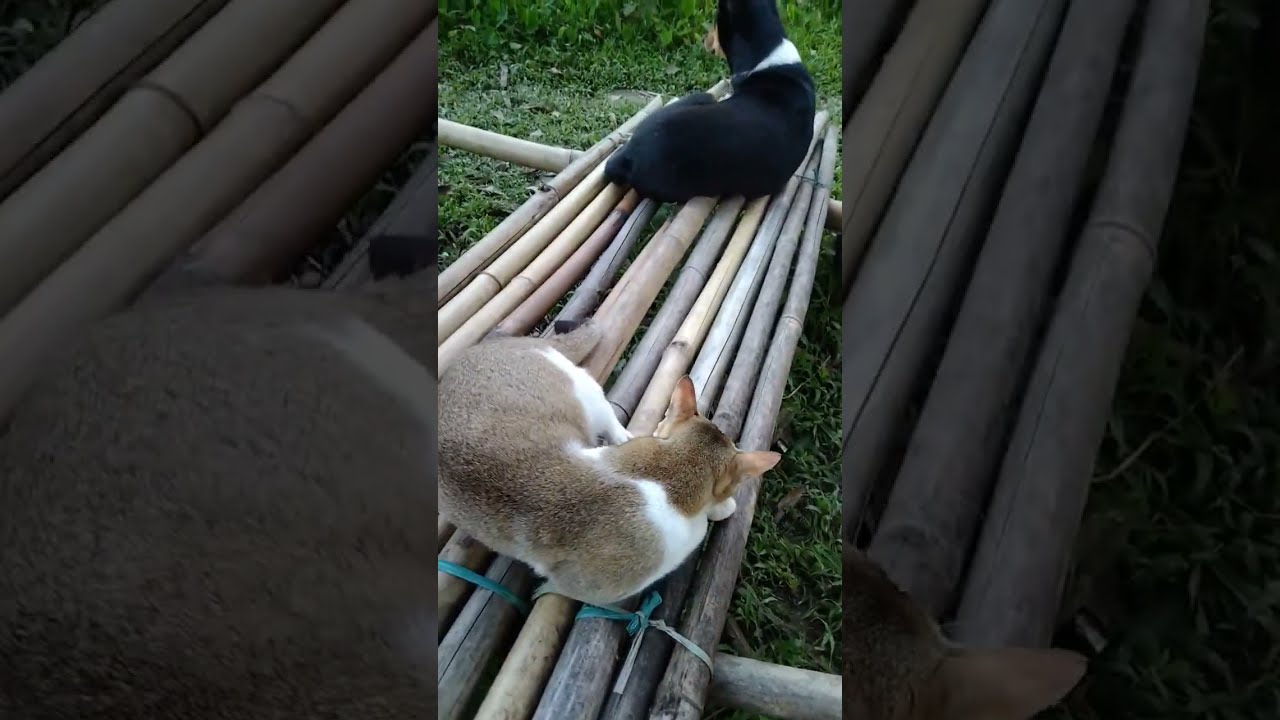In the image, two animals—a tan and white cat and a black and white dog—are laying on a homemade bench constructed from bamboo poles fastened together with rope or twine. The structure, resembling a raft, is positioned over a lush, green grassy area. Both animals are facing away from the camera, with the cat situated closer to the viewer and appearing to be asleep, while the dog is positioned further back. The setting appears to be an outdoor area, perhaps a well-kept backyard by a lake, and gives off an earthy, jungle-like vibe with rich green and brown tones. The bamboo structure occupies most of the image, and there is some greenery visible in the background. The image also has a split-screen effect, showing a close-up of part of the cat's body on the left and the cat's head and one ear on the right, enhancing the overall composition.